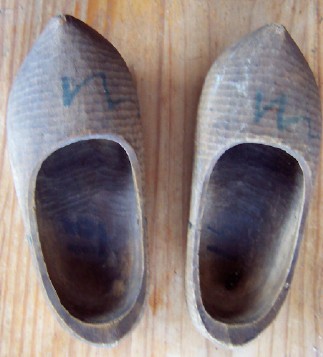This photograph is a close-up, top-down view of a pair of clogs placed side by side on a well-worn wooden surface. The wood underneath features vertical grains and is light-colored, contrasting with the medium to dark shades of the clogs. The clogs themselves are rather primitive in design, appearing retro or even ancient in style. They are slip-on shoes, lacking laces, and have a rounded base with a pointed tip at the top. The exterior of the clogs is light brown, while the insides are a much darker shade, almost black. Each shoe bears a distinct marking on the front toe area in blue; the left shoe has what looks like the letter 'n', and the right shoe features additional characters, possibly spelling out "n-easy". The photograph captures just the shoes, emphasizing their size and design details.